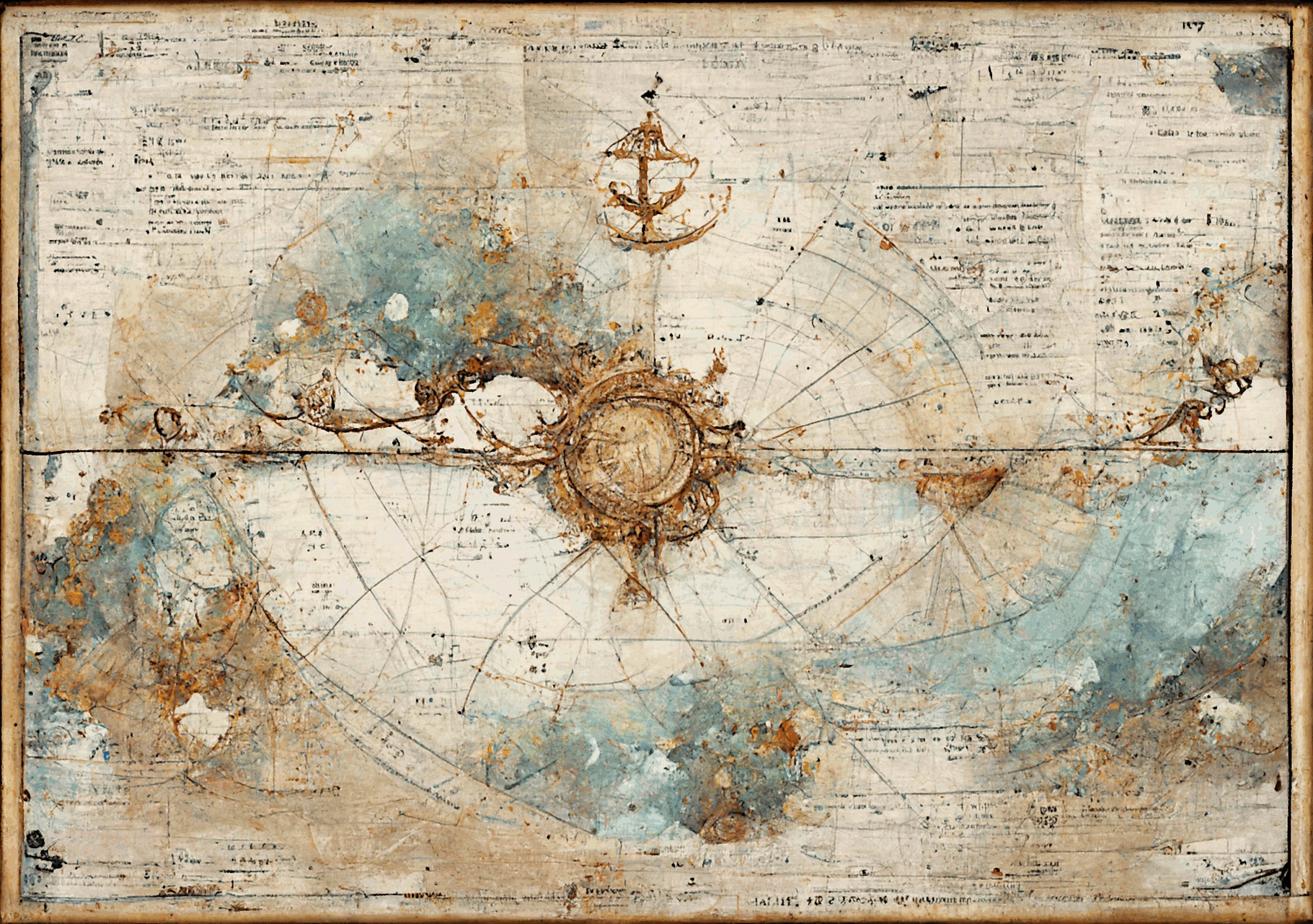This image portrays a rectangular, sepia-toned, antique-looking map that appears quite worn and abstract. Central to the map is a distinct circle featuring a lot of gold, potentially indicating a treasure site often associated with pirate lore. The map is rich in intricate and detailed lines with various features. Along the top, there's extensive writing, albeit hard to read, and on the top right, some numbering is visible. Above the central circle, there seems to be an anchor or a boat shape. Blue and bronze rust-colored splotches create a wave-like effect, particularly prominent in the bottom hemisphere and mid-center left. Despite these detailed elements, the map retains an abstract quality, making certain specifics challenging to discern at first glance.